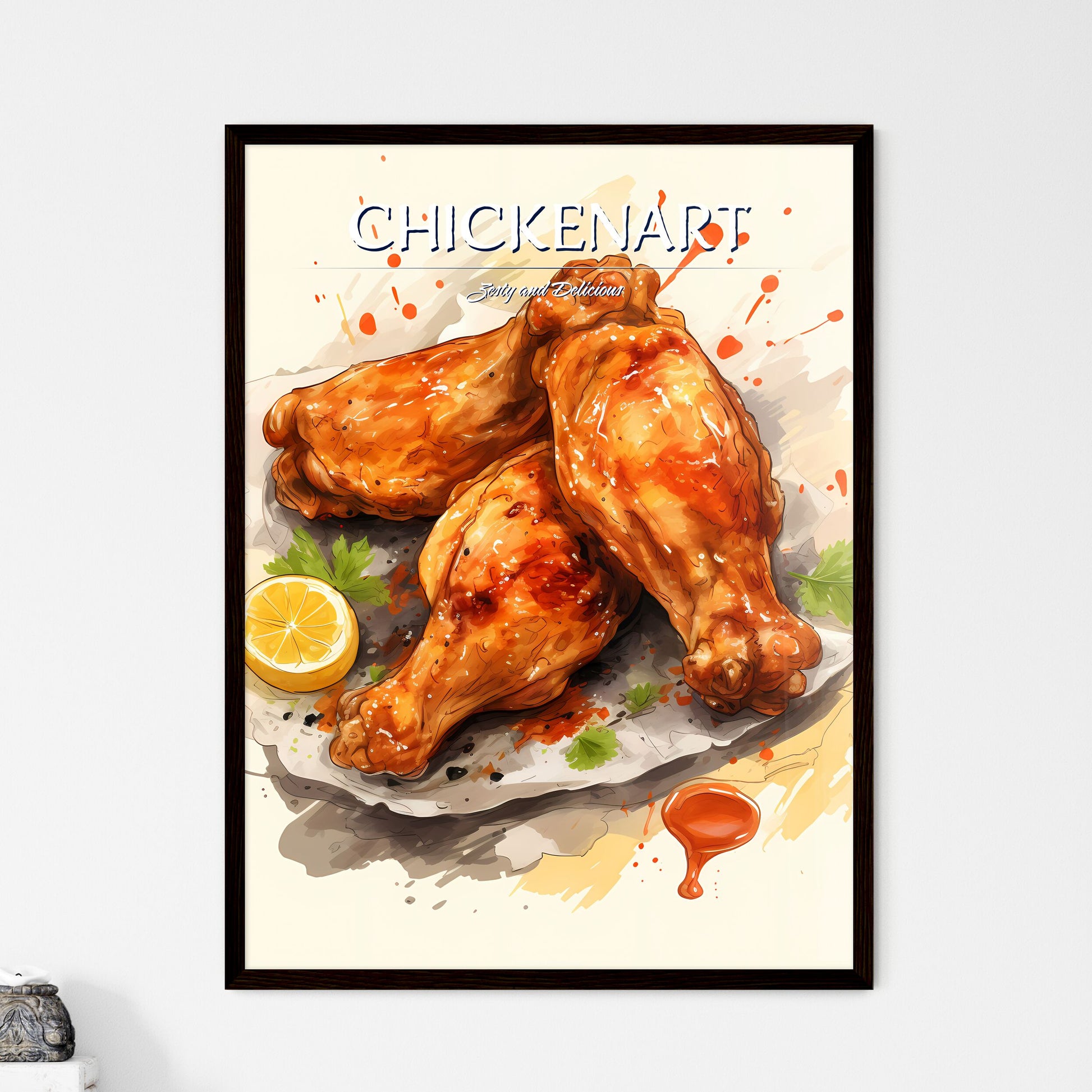The image depicts a white wall with a small shelf in the left-hand corner holding a gray pot. Dominating the right side of the picture is a rectangular black-framed art piece titled "CHICKEN ART" in bold white capital letters. Below this title is an underlining line, followed by the phrase "salty and delicious" in cursive. The artwork showcases three chicken wings, possibly legs or thighs, coated in a glistening honey barbecue sauce. These wings rest on a white plate along with a circular slice of lemon and some greenery, likely parsley. The background of the art is white, with artistic splatters of barbecue sauce extending beyond the plate and even appearing to splash onto the surrounding frame area. Additionally, an abstract splotch of barbecue sauce spills onto the tablecloth in the bottom right corner, further emphasizing the messy yet appealing presentation of the dish.